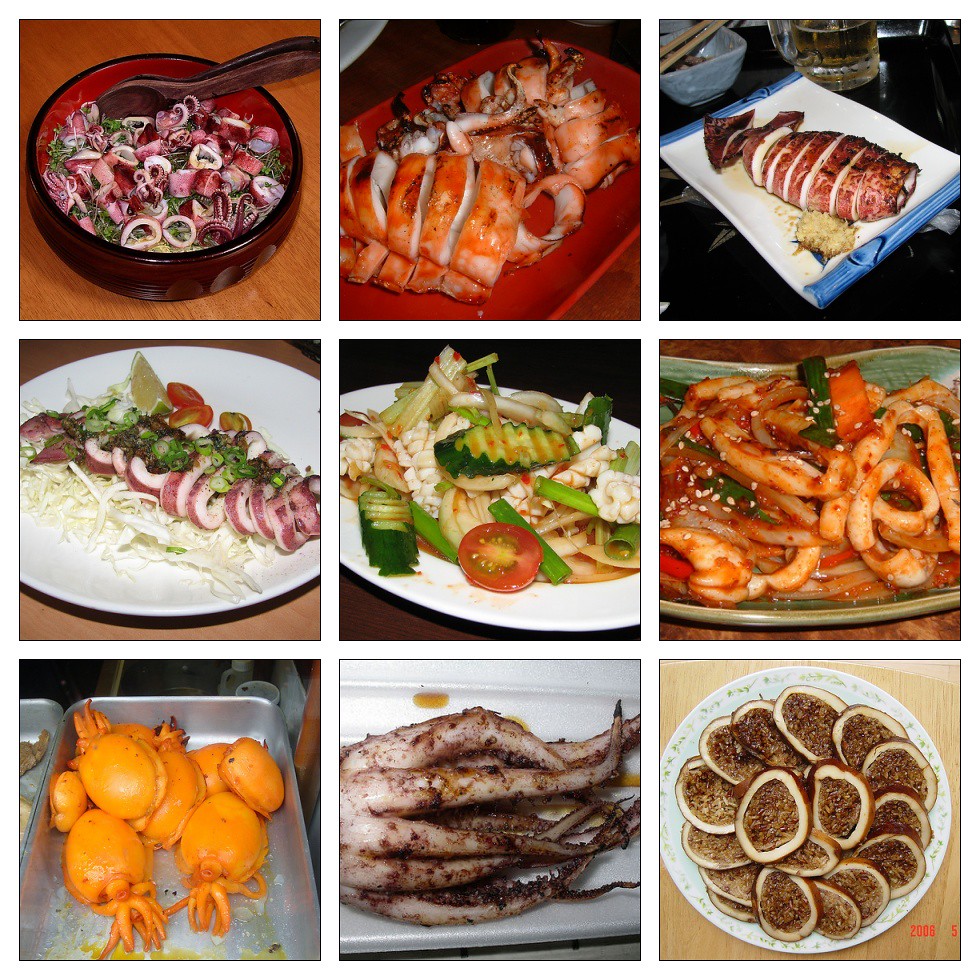The image is a color photograph split into a grid of nine smaller images, arranged in three rows and three columns, with equal white lines running through the divisions, giving a clean and structured layout. Each smaller image is encased in a thin black border. Predominantly depicting seafood dishes, the photograph showcases a variety of vibrant and appetizing seafood creations. In the bottom left corner, a rounded rectangular metal pan holds bright orange crabs. The middle bottom image features a whitish squid, its tentacles extending to the right, adorned with a brownish seasoning or sauce. The top middle and top right images display a fish that has been sliced across its body into sections. Other images include dishes such as seafood salad on white plates, octopus surrounded by green lettuce in a red bowl, and more brightly colored seafood varieties, all set against diverse backgrounds including wood surfaces and metal pans. A date stamp in orange, partially visible in the bottom right-hand corner, reads "2008," subtly marking the capture of this enticing spread of seafood delights.